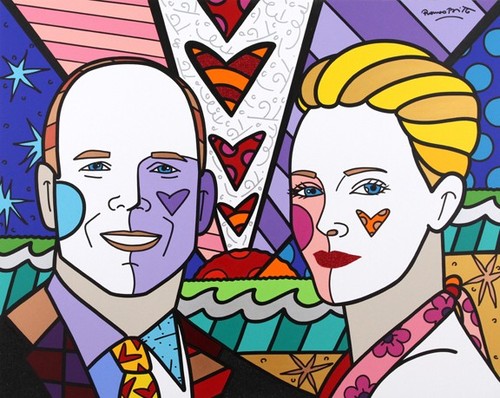This vibrant, pop art-style image vividly depicts an anthropomorphic cartoon-like man and woman set against a loud and bright background teeming with geometric shapes and colorful rays radiating from a central orb. The man, positioned on the left, has a distinctive two-thirds white face with a purple heart on his cheek, short brown hair, blue eyes, brown eyebrows, and is smiling. He's dressed in a multi-colored collared shirt, jacket, and tie. His female counterpart on the right is shown in partial profile with green-golden hair pulled back, blue eyes, an orange heart on her left cheek, and a red circle on her right cheek. She wears a white top that features a colorful scarf or collar. The background teems with multicolored shapes and patterns, including hints of green and blue waves suggestive of beach sand, woven together in a rich tapestry of orange, red, yellow, blue, green, purple, and pink hues, adding to the dynamic, cartoonish quality of the artwork.